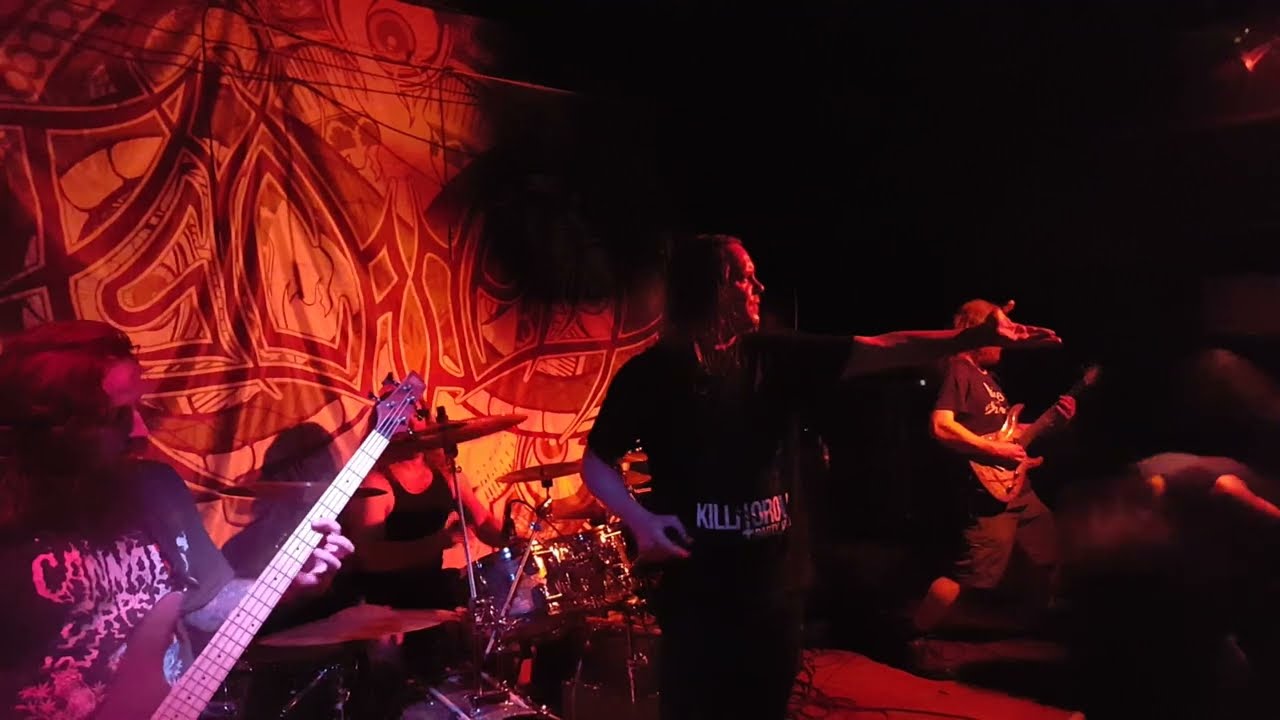The image depicts a live band performance, possibly a concert or a practice session, characterized by a dark ambiance with red lighting illuminating the scene. Central to the image is the lead singer, a man in his 50s with long hair, dressed in a black t-shirt and black slacks. His t-shirt has a fanny pack or belt across it, inscribed with the word "Kill" and possibly more letters. He stands in the center of the stage with his right arm by his side, likely holding a microphone, and his left arm reaching out as though trying to connect with someone. Behind him, a large curtain decorated in brown, cream, orange, and yellow tones forms the backdrop, adding to the visual appeal. To his left stands a guitar player with dark hair, wearing a black t-shirt featuring a white graphic, and playing an electric guitar. To his right, another guitarist, distinguishable by his beard and black t-shirt with indecipherable white lettering, also plays an electric guitar. Further to the right, there is a person, possibly an audience member, headbanging with their head down. Behind the lead singer, a drum set is also visible. The stage floor is adorned with a distinctive red carpet or rug, adding a pop of color to the otherwise dim setting.